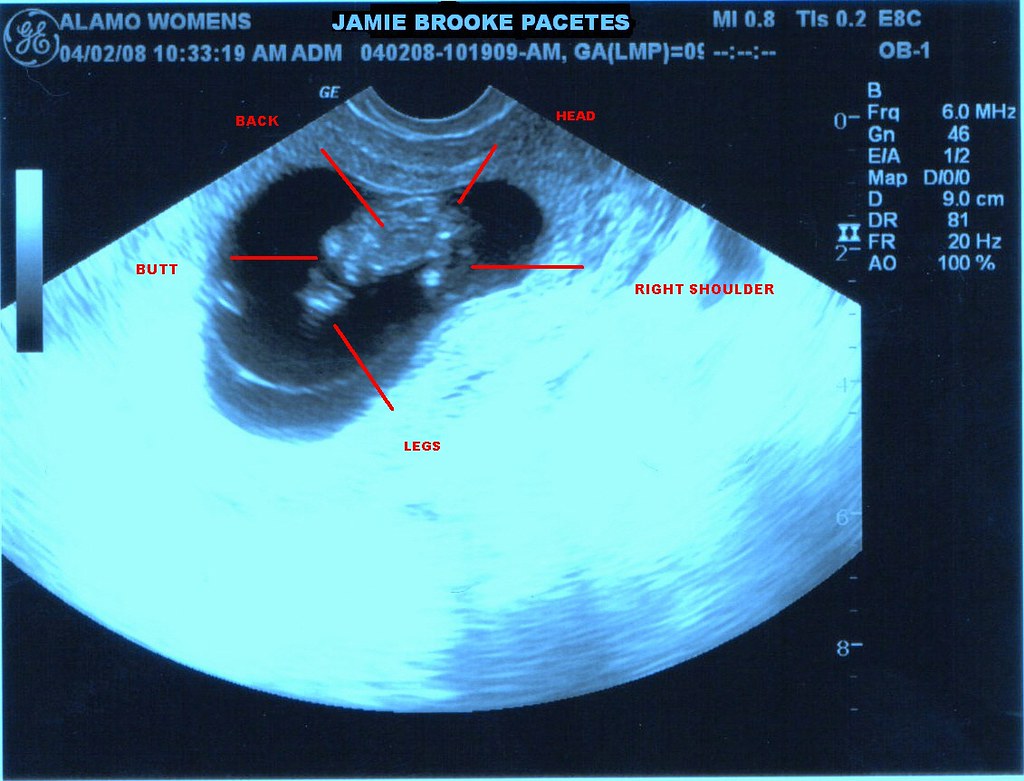The image is an ultrasound scan from a GE machine, taken at Alamo Women's on April 2, 2008, at 10:33:19 a.m. The scan is for the patient Jamie Brook Pasides. The image prominently features a distinctive, Doppler-shaped, V-like section highlighting the baby amidst a black background. There are red annotations marking key body parts such as the head, right shoulder, legs, butt, and back. Additionally, the scan includes various numerical and letter codes like 04-02-08-101-909-a.m., GA (LMP) = 09, MI.8, and TIS.2.